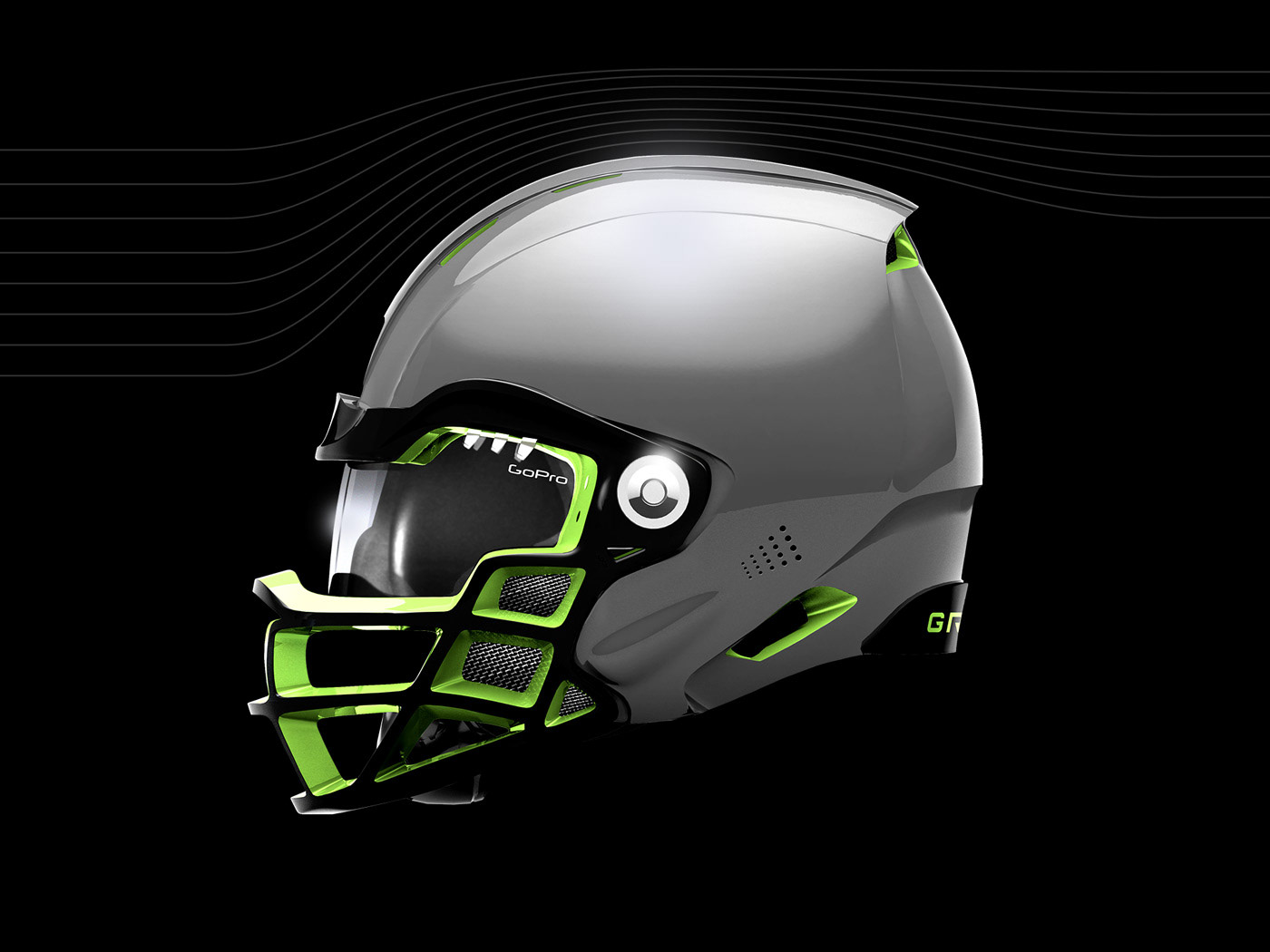The image features a large square format with a sleek black background and a series of thin, gray pinstripe lines that curve from the upper left to the upper right, totaling around seven or eight lines. Dominating the center is a futuristic-looking helmet, predominantly gray with neon green and black accents. The helmet, which could be used for sports such as football, lacrosse, or dirt biking, has distinct black face mask bars outlined in neon green, and several small vent holes near the ear area. Emblazoned across the eye goggles is the word "GoPro" in white lettering, while the back of the helmet features a partially visible black label with green text beginning with "GR." The helmet's design hints at advanced features, including built-in lights on the side and significant padding, making it ideal for high-intensity activities.